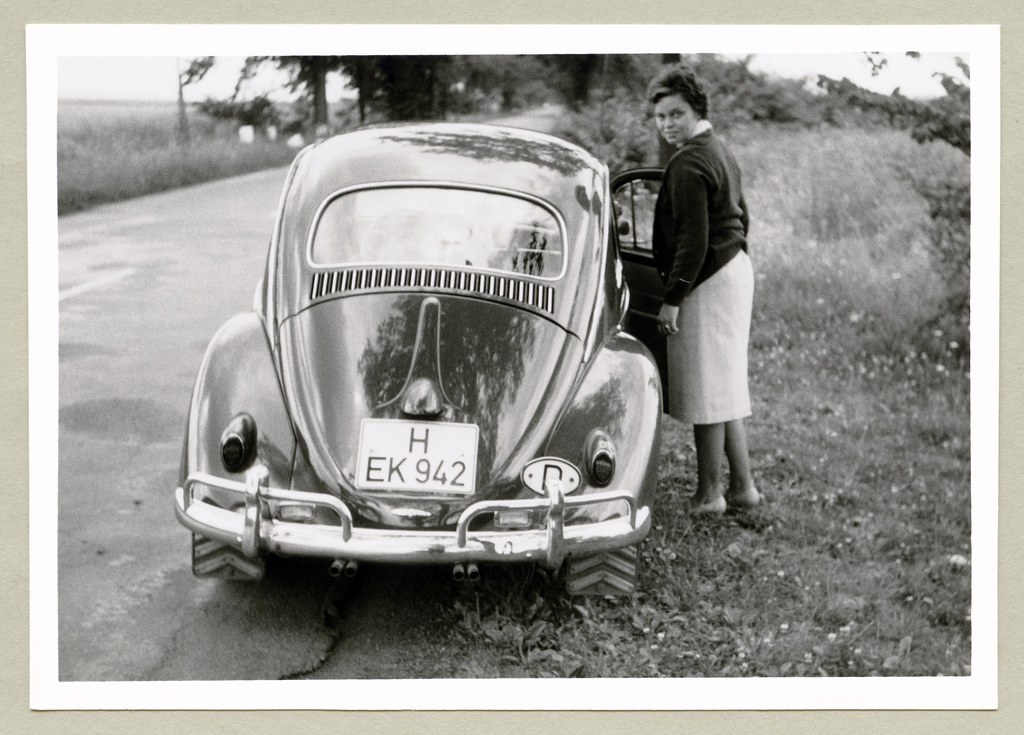A horizontally oriented black-and-white photo captures an outdoor moment featuring a vintage Volkswagen Beetle, parked on the side of a narrow country road. The shiny Beetle, with a silver back bumper, wide tires, and the license plate H-EK-942, is complemented by the rustic backdrop of trees and dried grass. A woman, dressed in a black sweater over a light-colored dress with a pencil skirt and dress shoes, stands with her back to the camera, her head turned towards the photographer. She is positioned next to the car with the passenger door open, as if about to get back inside. The scene is peaceful and captures a sense of timeless elegance amidst the simplicity of nature.